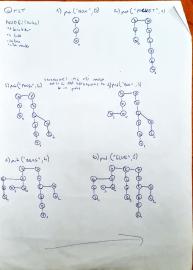This image is a low-quality, out-of-focus photograph of a white piece of paper. The paper is very small in the photo and appears to have a slight dog-ear fold in the upper right corner, revealing a dark brown surface behind it. The paper is filled with various handwritten notes in blue ink, though the text is too small to be legible. In the top right corner, there are four distinct pieces of writing. Adjacent to that, another segment of writing features three small, connected circles beneath it. In the upper left corner, additional notes are written, with a chain of ten small circles linked by a line underneath. The center of the paper showcases two lines of blue ink writing, followed by two diagrams consisting of circles connected by lines. This pattern of diagrams repeats further down the paper, though with slight variations in the designs. At the bottom, a blue pen-drawn arrow points to the right.